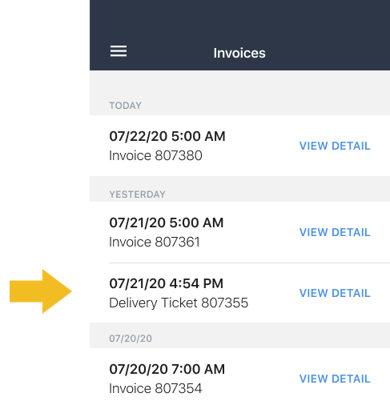The image depicts a webpage interface organized into several horizontal sections, each containing transaction details. At the top, there is a broad black band with three white bars aligned horizontally, which appear to be menu icons. Below this, a gray band displays the word "Today" in a slightly darker shade of gray.

The next section beneath this gray band is a white bar showing the date "07-22-20" followed by the time "5 a.m." and the label "Invoice 807380." To the right, there is a clickable "View Details" link in blue.

Further down, another light gray band reads "Yesterday" in darker gray text. Directly below, a white bar presents "07-21-20 5 a.m., Invoice 807361" with another blue "View Details" link beside it. Following this, another white bar notes "07-21-20 4:54 p.m., Delivery Ticket 807355" with an adjacent blue "View Details" link.

The subsequent gray band marks the date "07-20-20." Below it, a white bar states "07-20-20 7 a.m., Invoice 807354," accompanied by a similar blue "View Details" link. 

On the left side of the page, there is a golden yellow, computer-generated arrow directing attention to the "Delivery Ticket" entry.